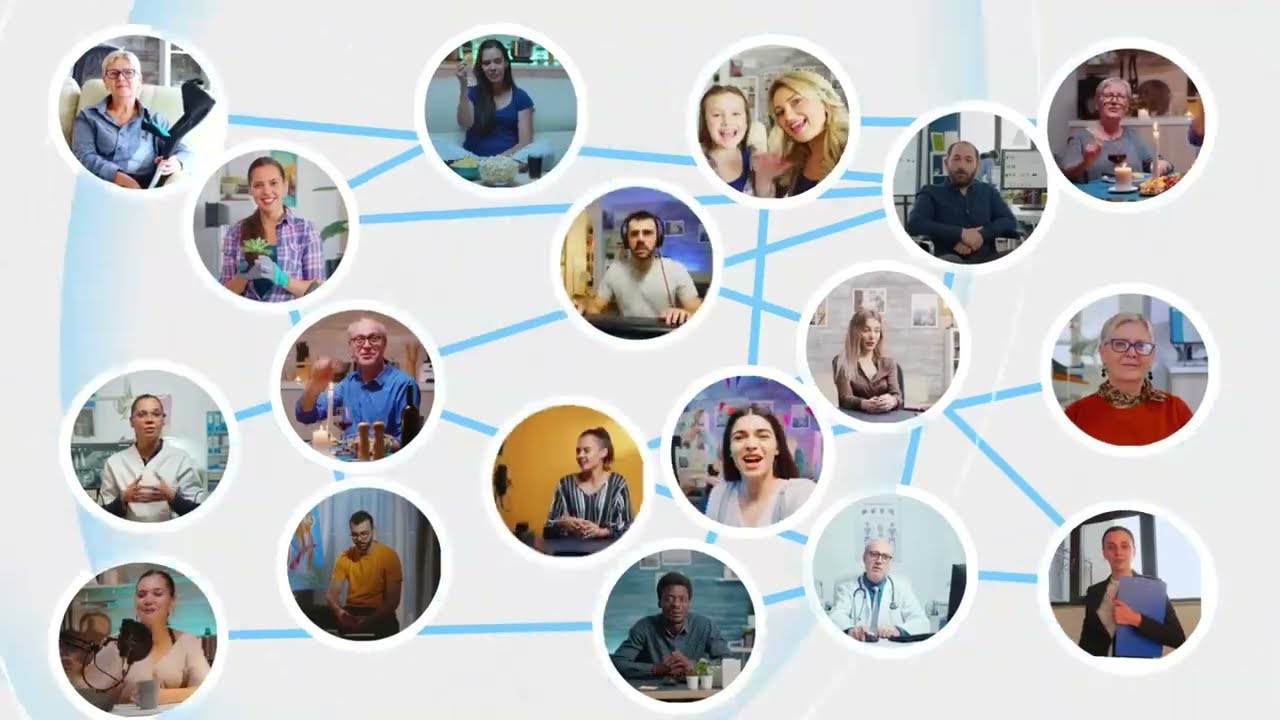This image is a detailed graphic set against a very light gray and soft blue background, featuring approximately 15 or slightly more white bordered circles, each containing a different person’s photo from the waist up. The subjects vary widely, including an older woman in a blue shirt on a white couch, a 20-something man in a white t-shirt at a computer keyboard with headphones, a doctor in a lab coat, and a florist in a purple patterned shirt holding a flower. Some circles depict two people, such as a possible mother and daughter duo. These circles are interconnected by blue lines, hinting at a network or relationship analysis, reminiscent of a family tree. No textual explanation is provided to clarify the context, but it visually illustrates various individuals connected through these blue lines, possibly indicating degrees of connectedness or interactions among them.